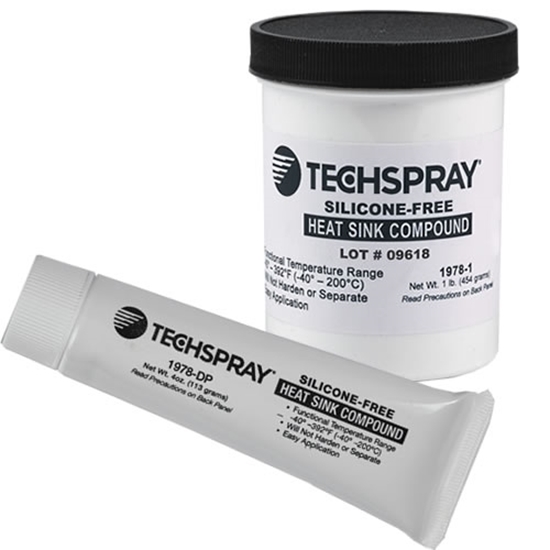The image depicts two Techspray products: a cylindrical jar and a tube of ointment. Both containers are primarily white with black text and are labeled "Techspray Silicone Free Heat Sink Compound." The jar, which is larger and has a black lid, details a net weight of one pound, a lot number 09618, and provides information regarding its temperature range, hardening properties, and usage precautions. Meanwhile, the smaller tube, positioned below the jar, also features a white body but with a matching white lid. It similarly includes product details, indicating a net weight of four ounces and additional temperature information. The labels on both containers display a round circle with white lines next to the Techspray logo. The photostyle presents a straightforward and clear focus on these products, emphasizing their shared design and informational content.